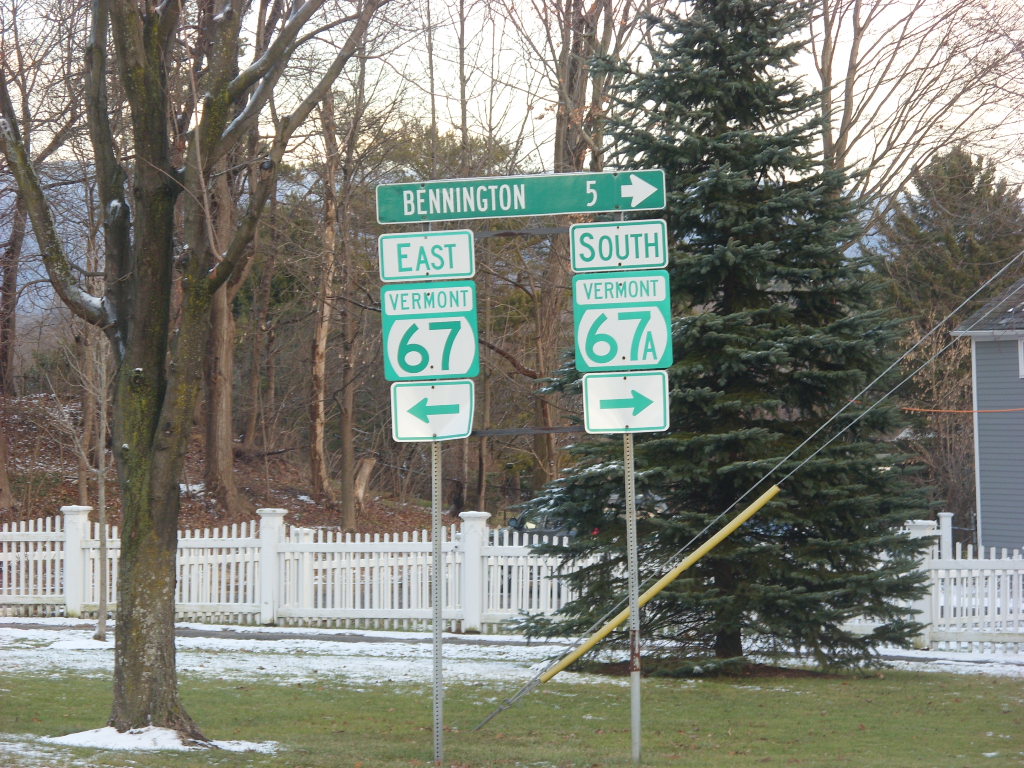This image features two directional road signs mounted on slender poles. The top sign points to the right and reads "Bennington, 5 miles," while the sign below it directs left and says "East Vermont 67." Positioned further down the post on the right side is another sign indicating "South Vermont 67A" with an arrow pointing right. In the background, a yellow, elongated cable protector encases a wire, adding a splash of color. The foreground is graced by a striking blue spruce tree, contrasting beautifully with its evergreen foliage. A charming white picket fence runs behind, punctuated by periodic pillars for support. Additional trees populate the scene, including one near the signs that stands bare without leaves. A thin blanket of snow covers the ground, revealing patches of grass, creating a picturesque winter landscape. In the right background, a gray house adds a touch of domestic tranquility to the setting.